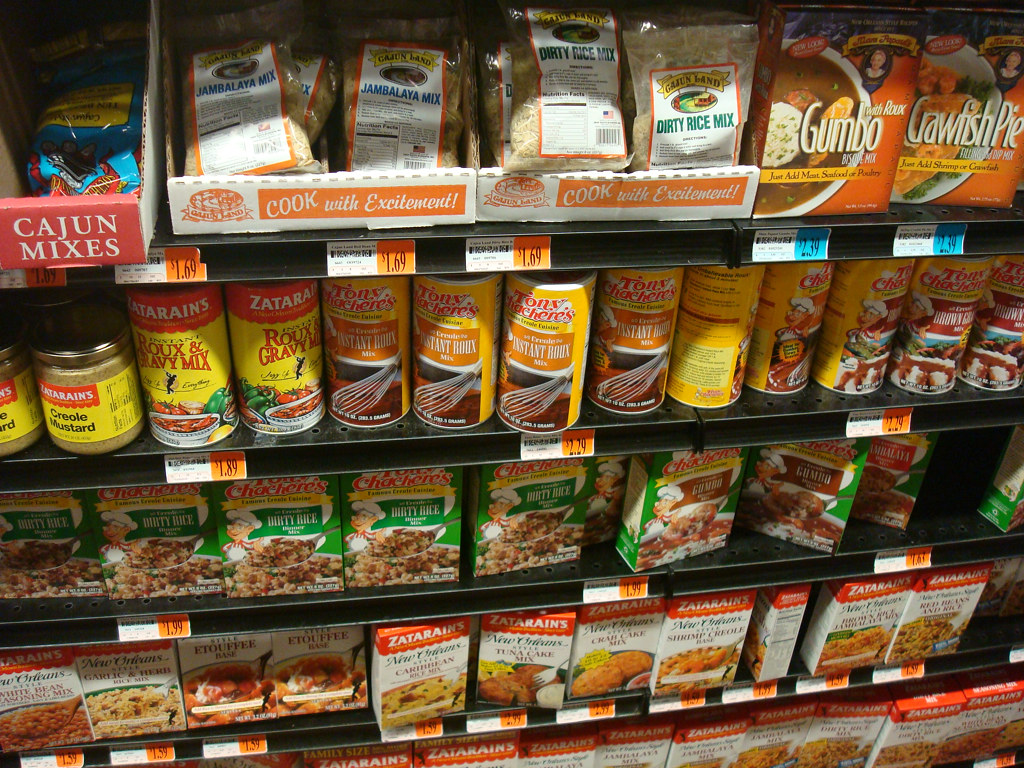This photograph captures the Cajun-style food aisle in a grocery store, showcasing multiple well-stocked shelves brimming with a variety of items. On the top shelf, vibrant plastic bags of rice mixes are prominently displayed, including varieties such as Dirty Rice, Jambalaya Mix, and Gumbo. These bags feature bold color schemes of white, orange, and blue, making them easy to identify. 

The next shelf down is lined with an assortment of mustards and gravy mixes, organized in canisters of various sizes. These items are encased in packaging bearing dominant hues of yellow, red, and mustard, creating a visually cohesive display. 

Descending to the third shelf, boxes of Dirty Rice take the spotlight. These packages are adorned with a playful cartoon chef on the front, set against a green background that highlights the brownish rice and red writing, making the product both appealing and easily distinguishable.

Finally, the bottom shelf presents an array of crab cake mixes from the brand Zatarain's. These are housed in white boxes with prominent red labels and appetizing food imagery, enticing customers with their culinary potential.